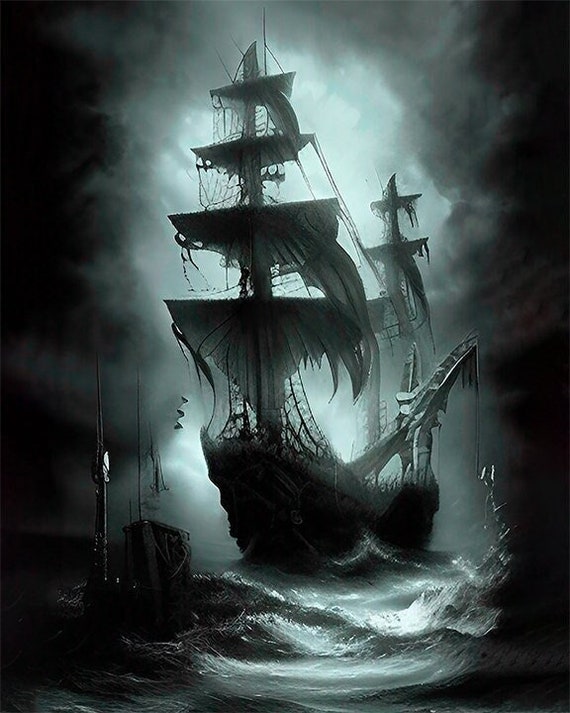The image is a detailed, monochromatic digital artwork of an ancient ship, reminiscent of those from the 1500s or 1600s, battling a tempestuous sea. Positioned in the center, the ship displays numerous tattered sails billowing wildly in the fierce storm, giving it an eerie, haunted appearance. The wooden structure of the ship itself seems jagged and spooky, enhancing its ghostly aura. The ocean beneath is depicted with high, crashing waves, illustrating the rough seas. In the bottom left corner, there's a dark, indistinct object with a spiky top, possibly another partially obscured ship, though its direction is unclear. Above, the sky is densely clouded, with some clouds illuminated as if by moonlight or a diffuse glow, adding to the dramatic and eerie atmosphere of the scene. The image is primarily rendered in shades of black and white with light blue highlights, creating a ghostly ambiance, while the darker edges contrast sharply with the brighter, more intense center where the ship is located.